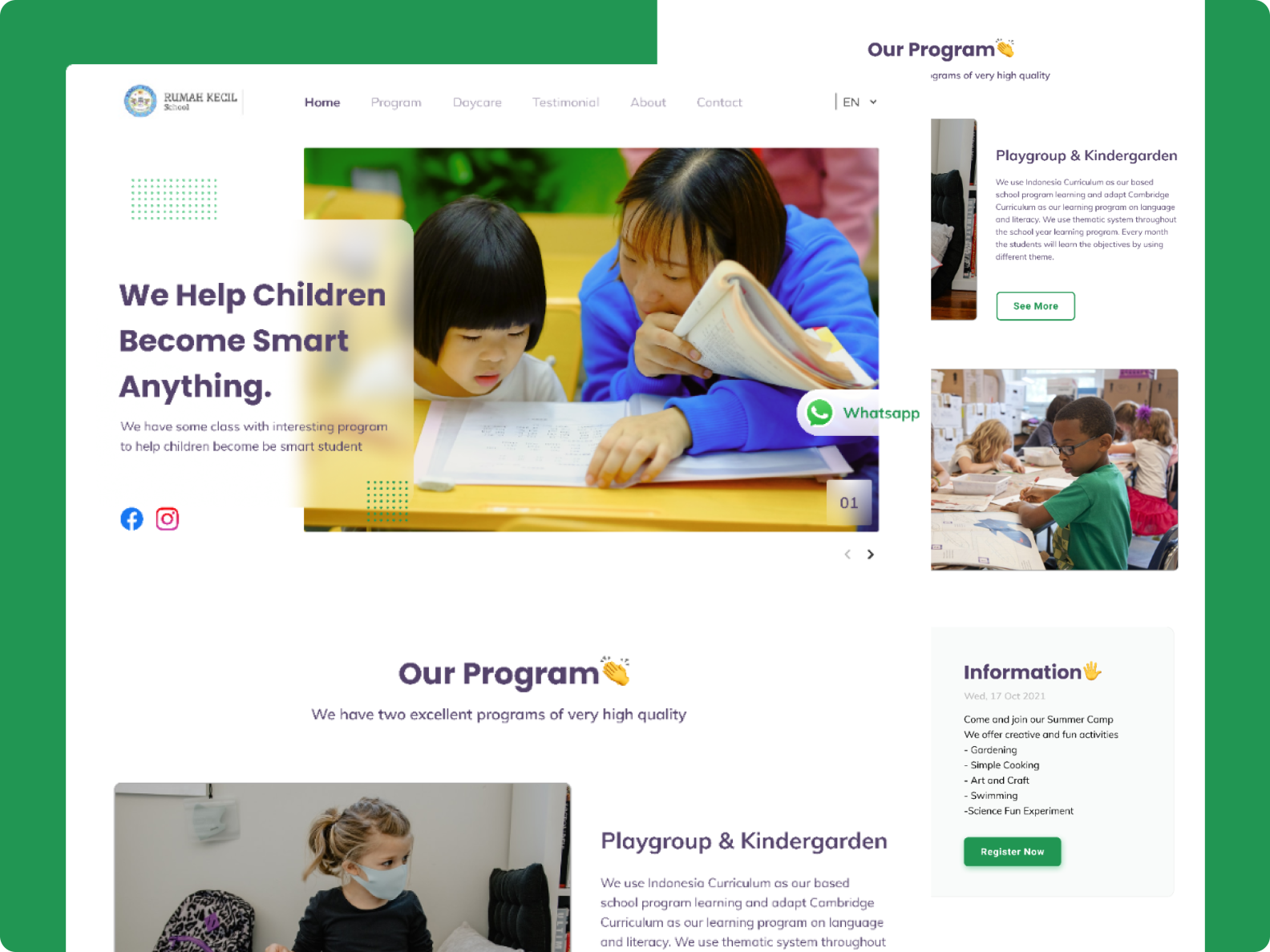### Detailed Caption for Website Screenshot:

The screenshot is of a website dedicated to children's education, characterized by a prominent white background encased in a medium green border that runs along the left side, right side, and halfway across the top. In the upper left corner, partially superimposed over a photograph, there's an image of an Asian child receiving assistance from a young adult teacher, who could also be a teacher's aide. Both individuals appear to be engaged in a learning activity.

Superimposed on this image is the text: "We help children become smart anything. We offer classes with interesting programs to help children become smart students." This text is likely translated from another language and reflects the educational theme of the website. Above this text, in small print, is the name "RUMAHKECIL," with additional tiny print beneath it, which is difficult to read.

In the upper right corner, in dark blue print, there is another text mentioning the high quality of their programs. Scattered along the right border is a text box labeled "Play Group and Kindergarten," accompanied by extremely small and tough-to-read text indicating that the website is related to educational activities in Indonesia. There is also a thumbnail image of children in a rural classroom setting, crowded around a table.

Below this, there is a text area with minimal blue print against a white background and a prominent "Register Now" button. Positioned towards the bottom center-right of the main section, the blue text reads: "Our Program," followed by: "We have two excellent programs of very high quality."

In the lower left corner of the screenshot, truncated at the bottom, is a photo of a young girl, approximately six to eight years old, with blonde hair and wearing a blue face mask. To the right of this image, the blue text states: "Play Group and Kindergarten. We use the Indonesian curriculum as our base school program and adapt the Cambridge curriculum for language and literacy learning." The text at the bottom is cut off, suggesting there may be additional information that is not fully visible in the screenshot.

This depiction offers deep insight into the educational services offered, highlighting a blend of local and international curricula aimed at fostering the development of young students.